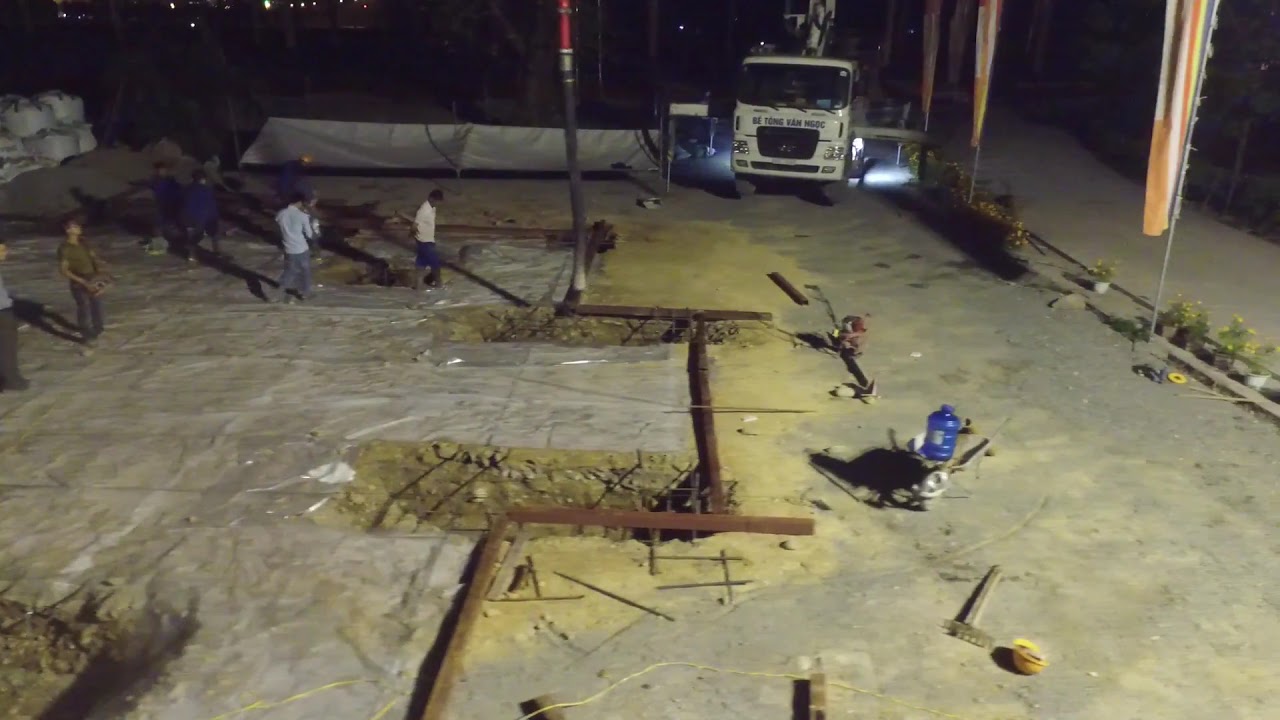This nighttime photograph depicts an active construction site bathed in artificial light, highlighting various details of the ongoing work. The ground is dotted with rectangular holes excavated by construction machines, each filled with metallic beams connected to stand-alone pipes rising vertically, likely forming the skeleton of a future structure. The site features a mix of plastic sheeting and concrete-covered areas, with crisscrossed boards directly on the ground. 

Construction workers are visible across the site, some inspecting and others actively working, while scattering various equipment including tools and a blue water jug. A yellow hard hat lies upside down in the foreground. To the right, a large expanse of gravel or cement is present, marked by tall metal poles adorned with orange flags. A white flat-fronted truck, resembling a semi, is parked further back on the right side, adding to the bustle of the location. Despite the dark sky, the scene is well illuminated by a source of bright artificial light, unseen in the image.